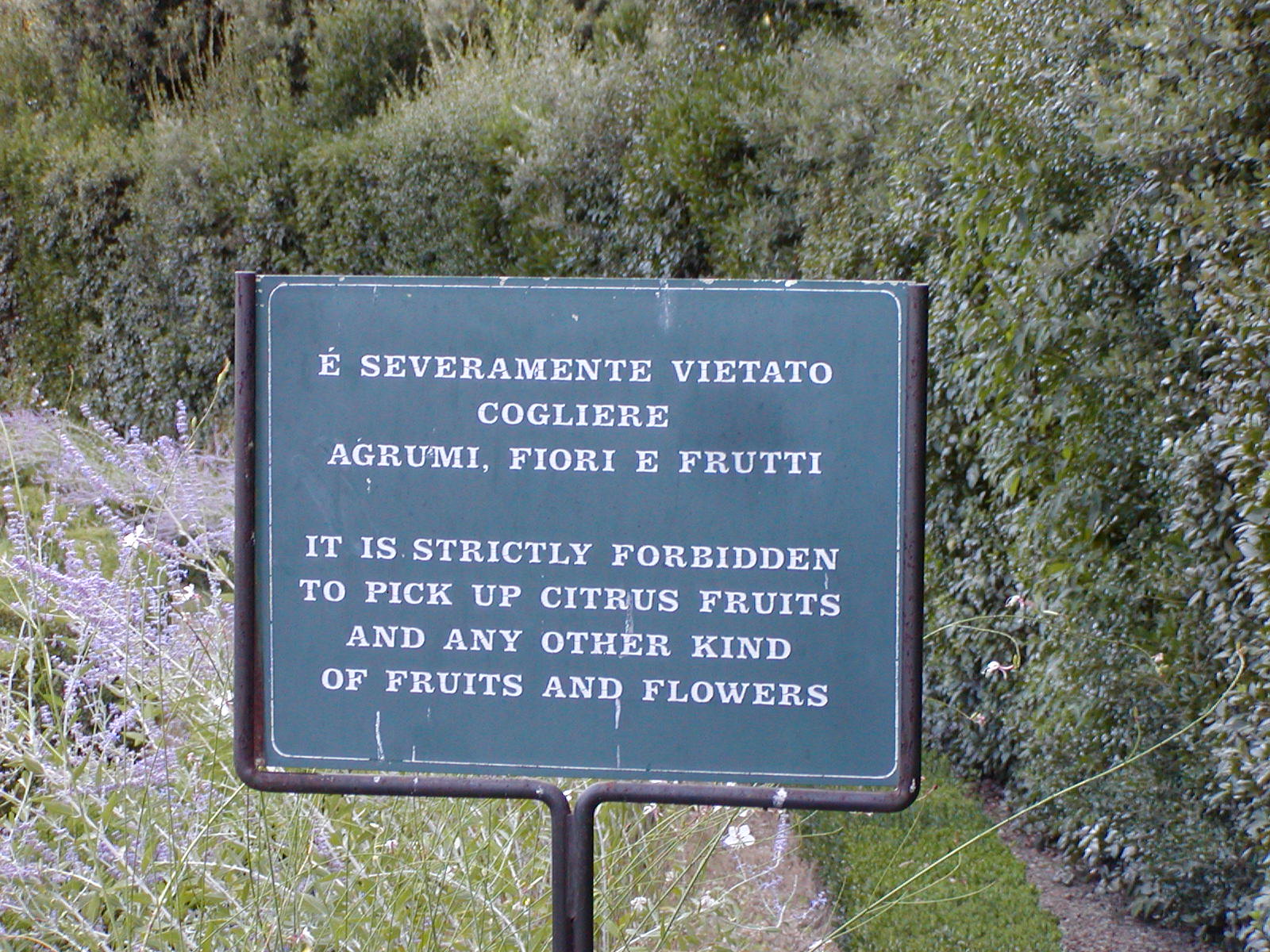The image features a nature scene with a central path flanked by diverse greenery. On the right, there's a dense barrier of thick green shrubbery, and on the left, wild grass, weeds, and purple flowers. This backdrop sets the stage for a prominent sign. The sign, a dark blue square with a black metal frame and pole, features text in both Spanish and English. The Spanish reads, "Severamente virutado coliogare agrumi fiori e frutti," while the English below states, "It is strictly forbidden to pick up citrus fruits and any other kind of fruits and flowers." Small lavender-colored flowers can be seen mingling with the bushes that form the background, adding to the vibrant natural setting.